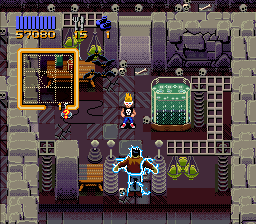This is a screenshot from a retro-style video game, captured from an aerial perspective inside a stone-built structure. The scene prominently features the stone-textured walls of the building running along the left and right sides of the frame. Towards the upper section of the image, a small doorway is visible, providing a sense of entry or exit within the game environment. In the upper left corner, there is a blue indicator line accompanied by the number "57090," likely representing the player's score or another significant game metric. At the center of the image stands the player's character, depicted as a small figure with spiky yellow hair, positioned as if ready to navigate through the game's challenges.